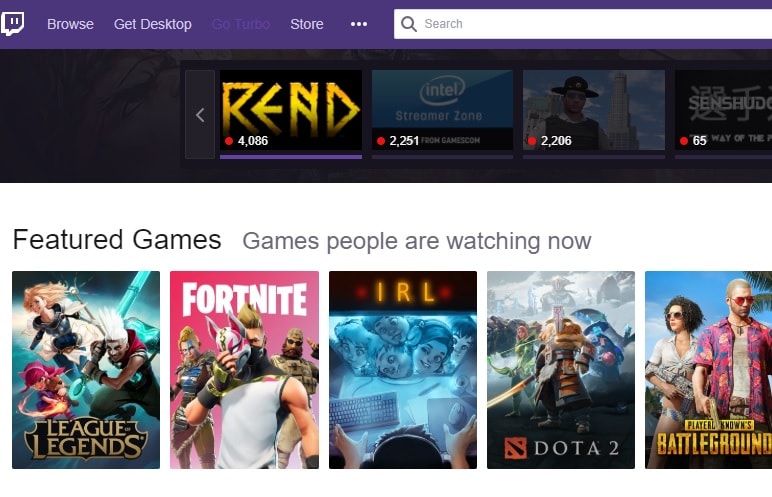This image is a detailed screenshot of a gaming store interface with a purple-themed header. At the top, a white search bar is prominently displayed, accompanied by various navigation options including "Browse," "Get Desktop," and "Go Turbo." Additionally, there are three horizontal dots signifying a menu, and a text label that reads "Rend Intel Streamers." The main section showcases several categories: "Featured Games" and "Games People Are Watching Now." Listed under these categories are popular titles such as League of Legends, Fortnite, IRL, Dota, and PlayerUnknown's Battlegrounds. Each game icon is accompanied by small red dots indicating the number of viewers, such as 4,000, although it does not display the number of active players. Graphics within the screenshot hint at in-game scenes, like characters battling in League of Legends and masked avatars in Fortnite. This interface provides a snapshot of trending games and current viewer engagement.